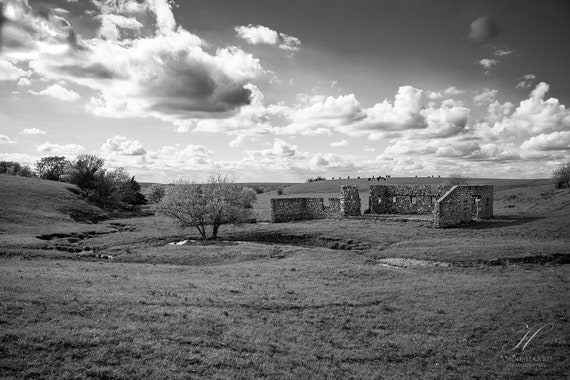This detailed black and white photograph depicts a serene, expansive countryside scene. Dominating the middle of the image are old, incomplete stone ruins or unfinished brick buildings that appear to have once been houses. The ruins, with their exposed foundations and missing walls and roof, evoke a sense of abandonment. Surrounding these structures, the scene is characterized by a lush grassy field with trees and bushes interspersed, particularly two small trees positioned near the buildings. A small creek gracefully winds through the grassland in front of the ruins, adding to the tranquil atmosphere.

The sky is filled with cumulus clouds against a grayish backdrop, indicating a cloudy day with darker overtones towards the top right. This professional, high-quality photograph, though absent of human presence, captures the timeless beauty of a secluded rural landscape. Text and a logo, partially highlighted by a cursive 'H', can be found at the bottom right corner of the photo.